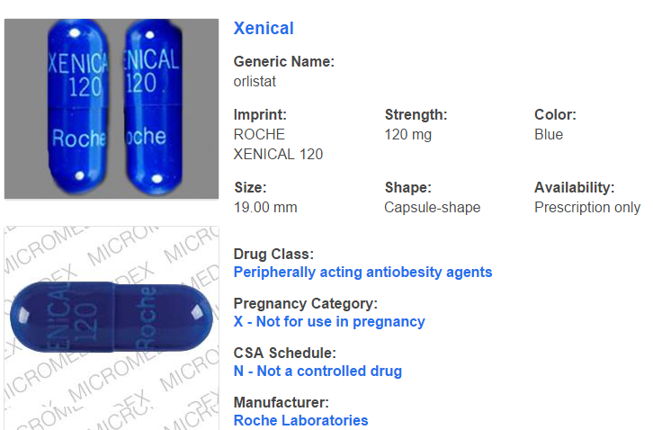This image is a cropped screenshot of a medication listing, featuring detailed visuals and information about the drug. On the left side of the image, there are two large square thumbnails showcasing the medication in capsule form. 

The first thumbnail, positioned at the top left, displays two capsules aligned vertically. The capsule on the left prominently shows the name of the medication, "Zenecal," at the top, and the manufacturer, "Roche," at the bottom. The second capsule provides a side view where the rest of the word "Zenecal" and "Roche" are visible. 

The bottom thumbnail offers a side view of a blue capsule lying on its side. 

A Micrometics watermark covers the background of the product photos. To the left of the thumbnails, the medication name, "Zenecal," is written in bold blue letters. 

Below this title, the listing displays various details about the drug: 
- Generic Name
- Imprint
- Strength
- Color
- Size
- Shape
- Availability
- Drug Class
- Pregnancy Category
- CSA Schedule
- Manufacturer

This screenshot has been cropped to focus on the essential elements of the medication listing.